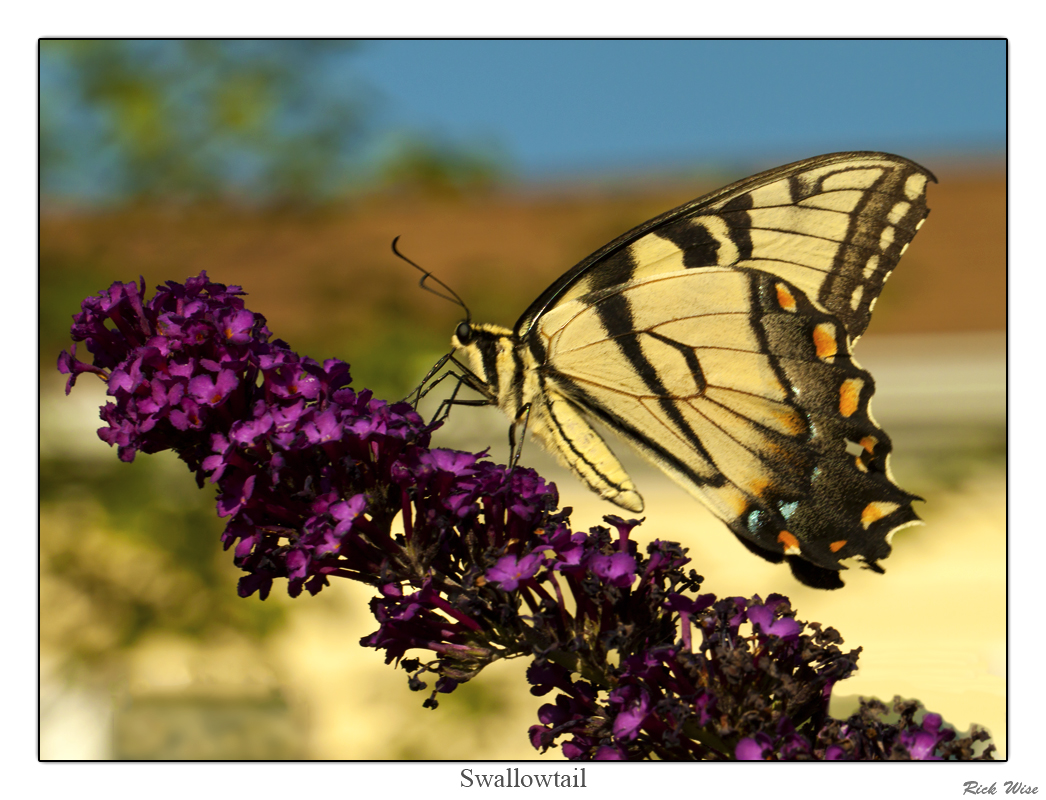This rectangular outdoor photograph, bordered in black as if framed, captures a vivid scene bathed in natural light. Though the background is softly blurred, hints of greenery, trees, and shrubs suggest a lush, vibrant setting. The photograph's focal point is a striking butterfly poised delicately on a flower. This butterfly, a Swallowtail, boasts yellow wings adorned with intricate black markings, with the tips of its wings showcasing a blend of yellow, orange, and black hues. The flower, elegantly elongated, comprises numerous tiny blossoms of a bright purple shade, while its stems reveal a nearly reddish tint. Below the photograph, the word "Swallowtail" is inscribed in black print, and in the bottom right-hand corner, the name "Rick Wise" is discreetly noted.